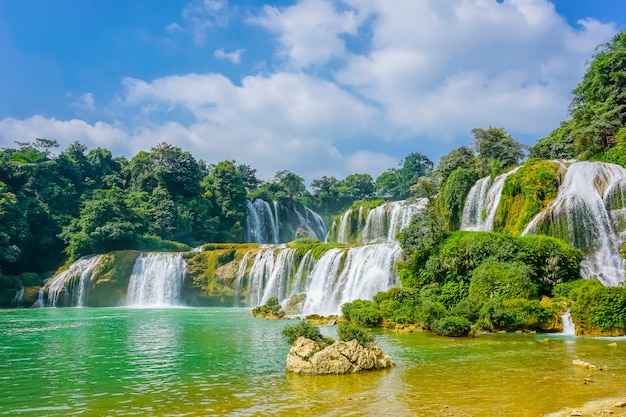This is an outdoor photograph capturing a serene, tropical landscape. In the forefront of the image, there's a shallow waterway with portions of brown ground visible beneath it on the right side, while the left side appears deeper and is tinged with a lush green hue. Scattered light brown rock formations punctuate the water, accentuated by patches of greenery growing atop. Dominating the middle and background are numerous cascading waterfalls, approximately eight, flowing over moss-covered rocks, creating a visually stunning, multi-tiered water cascade. The waterfall areas are enveloped by thick clusters of vibrant green trees and bushes, contributing to the dense, lush ambiance of the scene. In the distance, the towering trees boast dense foliage, lending further tropical character to the landscape. Capping this picturesque setting is a bright blue sky adorned with numerous fluffy, white clouds, adding a sense of calm and openness to the composition.